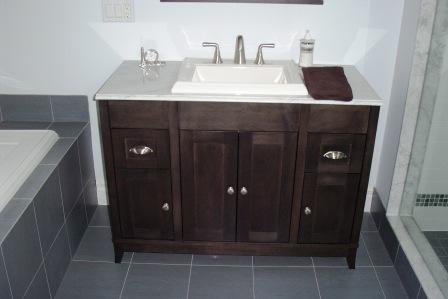The image showcases a well-appointed bathroom with a modern aesthetic. The floor and tub surround are adorned with square, gray tiles. On the left side of the image, there's a white jet tub, while the right side features a step-in shower with white walls and a tiny mosaic tile border at the base.

At the center of the image is a sink, encased in a dark-stained wooden cabinet. The cabinet features silver fixtures, including round silver knobs on the lower cabinet doors and scoop-type handles on the two upper drawers. On the countertop, which appears to be polished marble or granite, rests a chocolate brown towel. The countertop also supports a white enameled sink with matching silver fixtures.

Behind the towel on the right side sits a pump bottle of soap, while on the left side there's an ornamental crystal object, likely a ring holder. The very bottom edge of a mirror is visible above the sink, with a switch plate featuring two flat switches and two outlets positioned below it, over the cabinetry. Only the top corner of the white tub is visible, providing a glimpse of the luxurious bathing area.